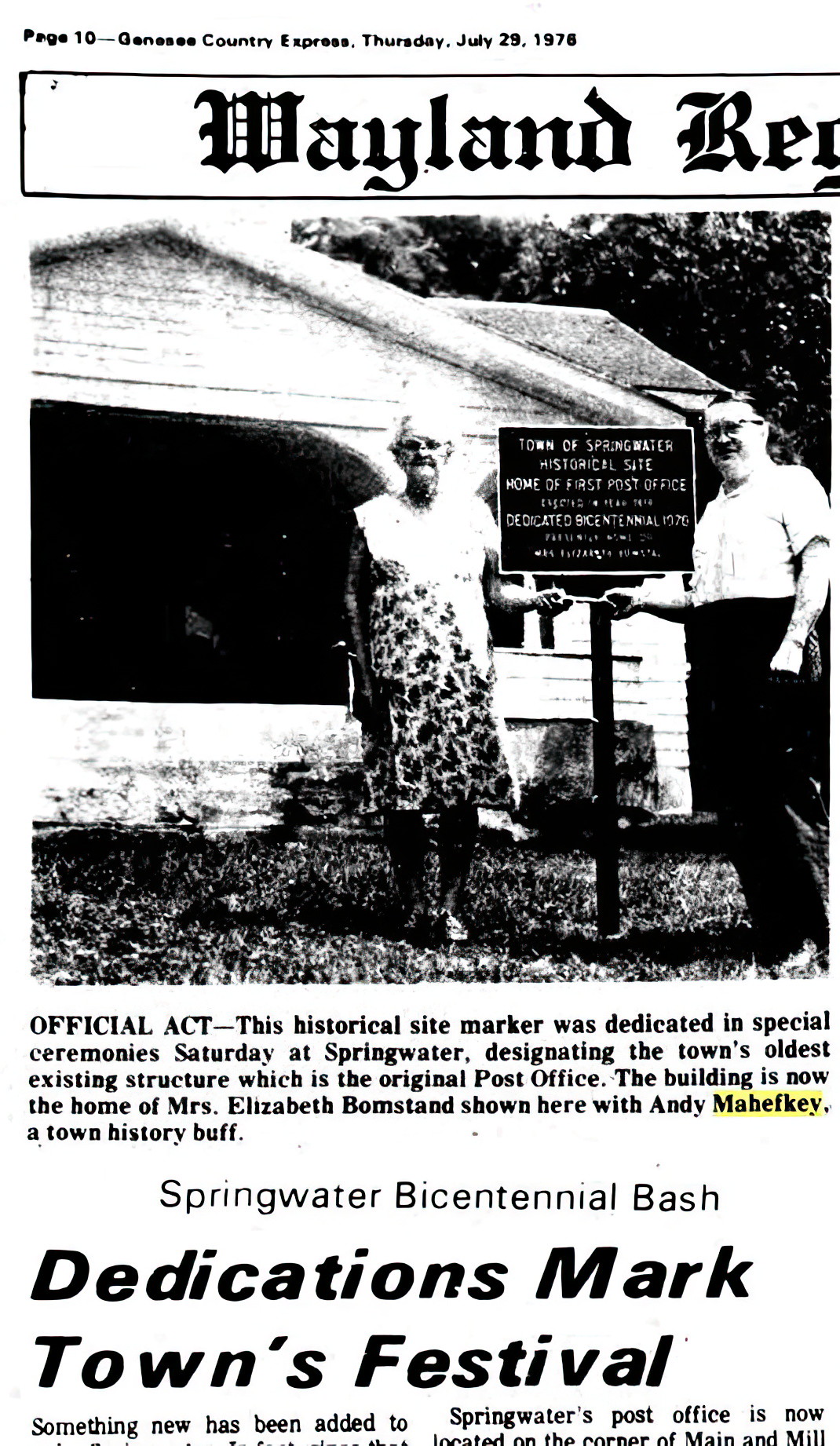This detailed black-and-white vintage newspaper clipping appears to be from page 10 of the Genesee County Express, dated Thursday, July 29, 1976. At the top, the partially cut-off headline reads, "Wayland, R-E-G." The main feature of this page is an overexposed photograph depicting an older couple, Mrs. Elizabeth Balmstad and Andy Mahefke, standing beside a historical site marker labeled "Town of Springwater Historical Site," with an old house in the background. The caption below the photograph states: "Official Act: This historical site marker was dedicated in a special ceremony Saturday at Springwater, designating the town's oldest existing structure, which is the original post office. The building is now the home of Mrs. Elizabeth Balmstad, shown here with Andy Mahefke, a town history buff." Andy Mahefke’s name is notably highlighted in yellow. Below this caption, another headline reads, "Springwater Bicentennial Bash: Dedications mark town's festival," followed by a paragraph that has been cut off.